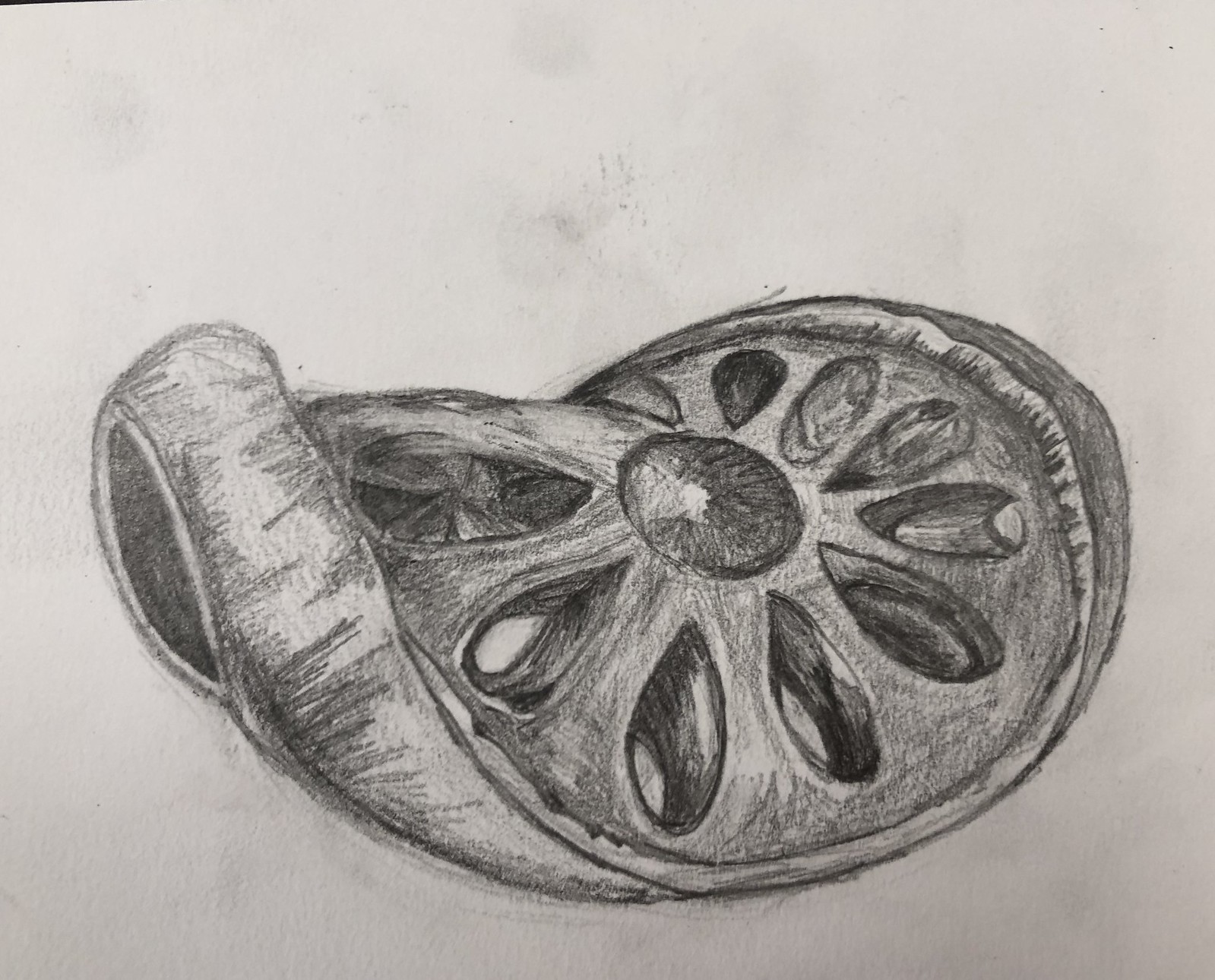This image is a detailed pencil sketch on white drawing paper, showcasing either a bent slice of fruit, like an orange, or a twisted hubcap, perhaps symbolic and open to interpretation. Sketched in graphite, the primary focus of the drawing is centered slightly lower on the page, where a round, central circle is depicted with darker shading. From this center, extends a series of teardrop or oblong shapes, resembling the holes of a lotus pod or the openings of a car rim, with about ten of these shapes visible. These elements are meticulously shaded to give depth and dimension, suggesting that the holes penetrate the object. The entire subject appears to be curved, as if bent or twisted over a pipe, giving it a morphed, dynamic quality. The white background contrasts sharply with the detailed shading, which is further accented by smudges from pencil lead, possibly from fingerprints or hands, adding to the artistic, in-progress feel of an art school assignment.